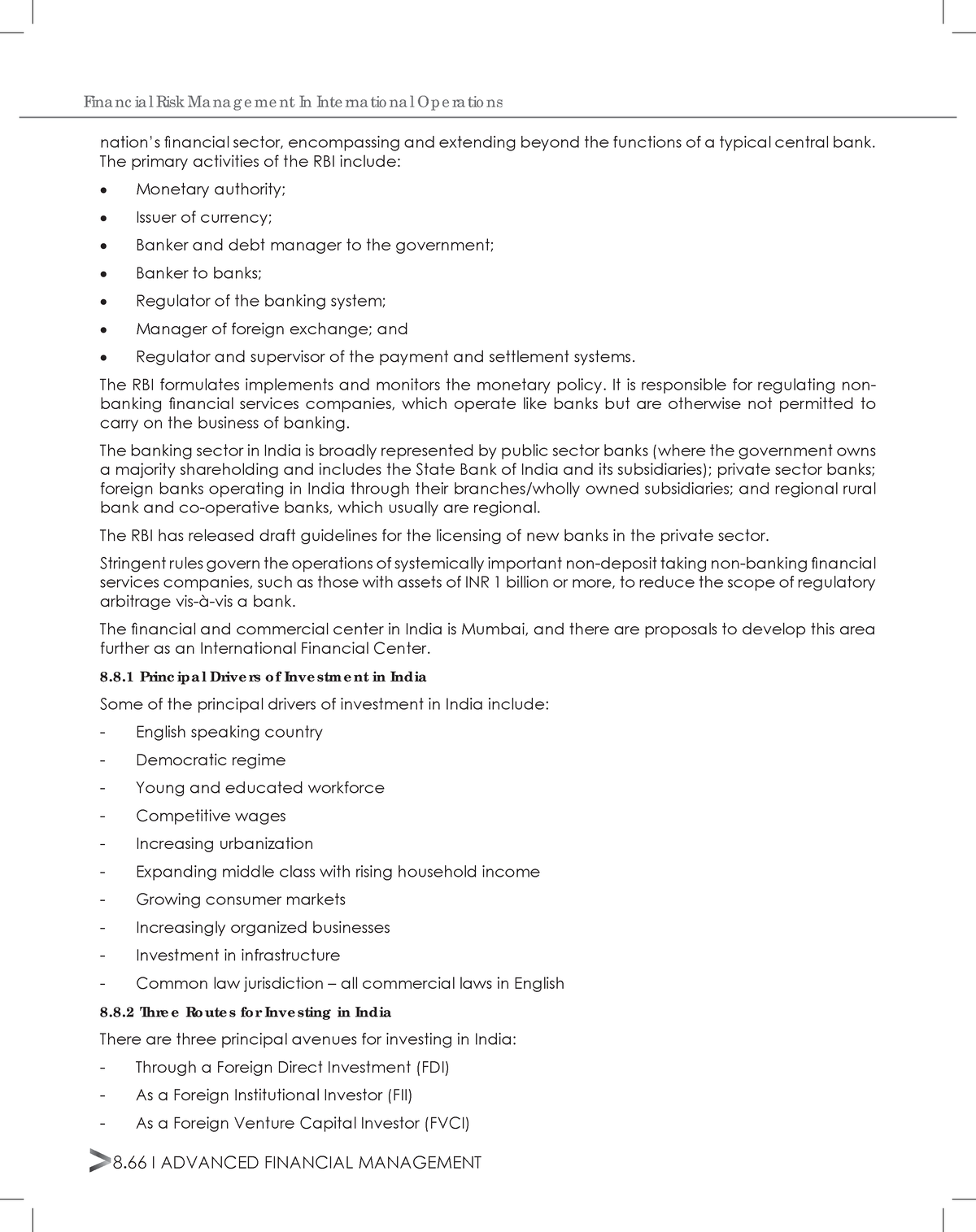**Caption:**

The image showcases a detailed document titled "Financial Risk Management in International Operations" displayed prominently in gray at the top. Below the title, there is an informative article detailing the extensive functions of a nation's financial sector, which go beyond the typical roles of a central bank. Specifically, it focuses on the Reserve Bank of India (RBI). 

The article elaborates on the key activities of the RBI, which include formulating, implementing, and monitoring monetary policy. Additionally, it outlines the RBI's responsibility for regulating non-banking financial services companies that operate similarly to banks but are not licensed to engage in banking activities.

A comprehensive overview of India's banking sector is provided, highlighting the public sector banks where the government holds a majority share. This includes the State Bank of India and its subsidiaries. The description also covers private sector banks, foreign banks operating in India through their branches or wholly-owned subsidiaries, and regional, rural, and cooperative banks that typically serve local areas.

Furthermore, the article mentions that the RBI has issued draft guidelines for the licensing of new banks in the private sector. These guidelines aim to enforce stringent rules for systematically important non-deposit-taking non-banking financial companies with assets of INR 1 billion or more, thereby reducing the potential for regulatory arbitrage in the banking sector.

There are additional bullet points and text providing further details, continuing the comprehensive coverage of financial risk management practices in international operations.